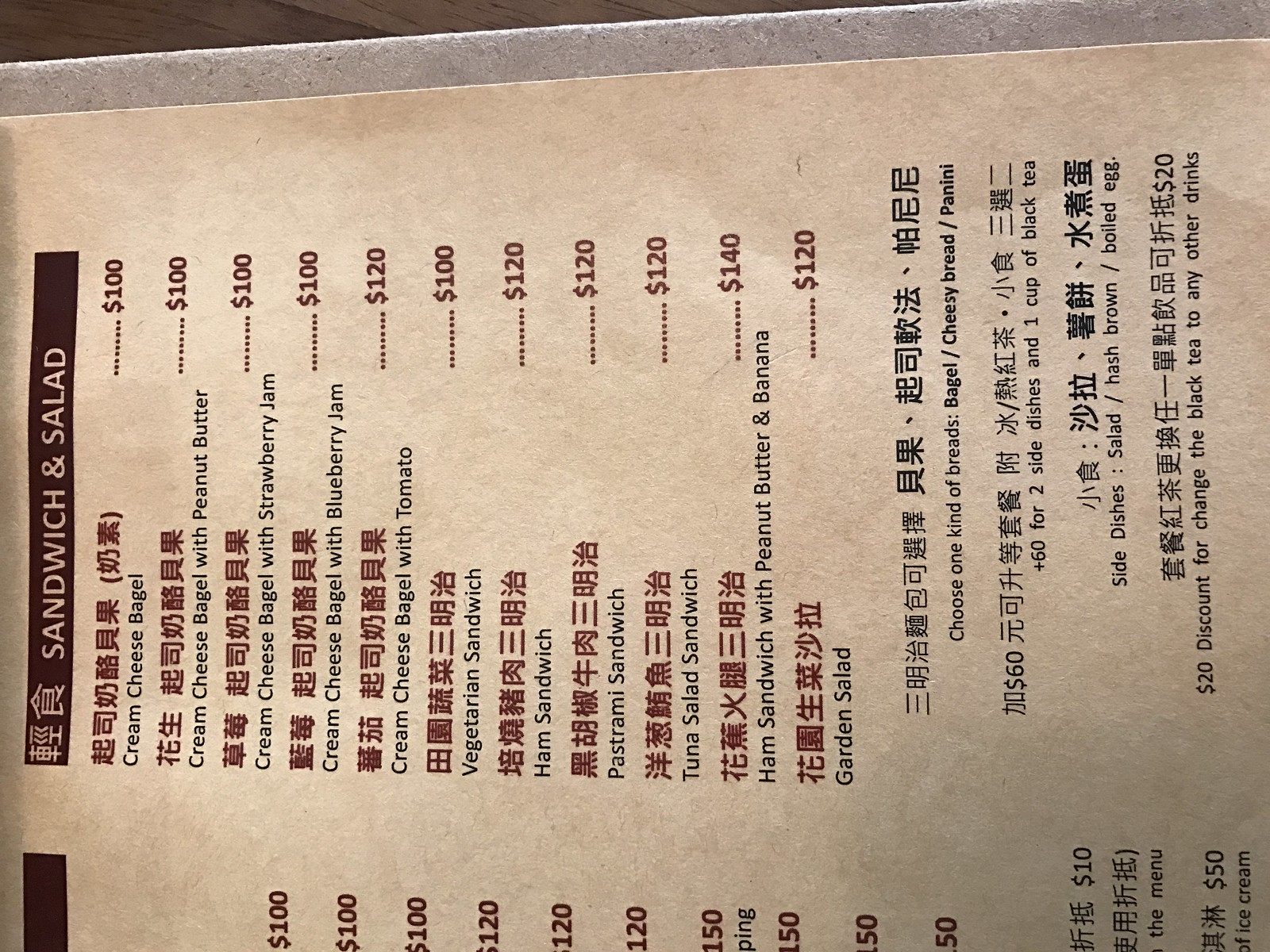The sideways-oriented menu displays a variety of sandwiches and salads, with headings at the top that include "Sandwich" and "Salad". The menu features several items listed with prices, albeit with a seemingly erroneous formatting where $1.00 is written as "$100"; this could be attributed to a translation or printing error, as evidenced by the accompanying Chinese characters.

**Menu Items:**
- **Cream Cheese Bagel:** $1.00
- **Cream Cheese Bagel with Peanut Butter:** $1.00
- **Cream Cheese Bagel with Strawberry Jam:** $1.00
- **Cream Cheese Bagel with Blueberry Jam:** $1.00
- **Cream Cheese Bagel with Tomato:** $1.20
- **Vegetarian Sandwich:** $1.00
- **Ham Sandwich:** $1.20
- **Pastrami Sandwich:** $1.20
- **Tuna Salad Sandwich:** $1.20
- **Ham Sandwich with Peanut Butter and Banana:** $1.40
- **Garden Salad:** $1.20

At the bottom of the menu, there are further details provided in Chinese, along with the following options and additional pricing:
- **Choice of Bread:** Bagel, Cheesy Bread, or Panini
- **Add-ons:** +$0.60 for two side dishes and one cup of black tea
- **Discount:** $0.20 off for changing the black tea to any other drink

This detailed breakdown ensures clarity and accuracy for potential customers navigating the menu.